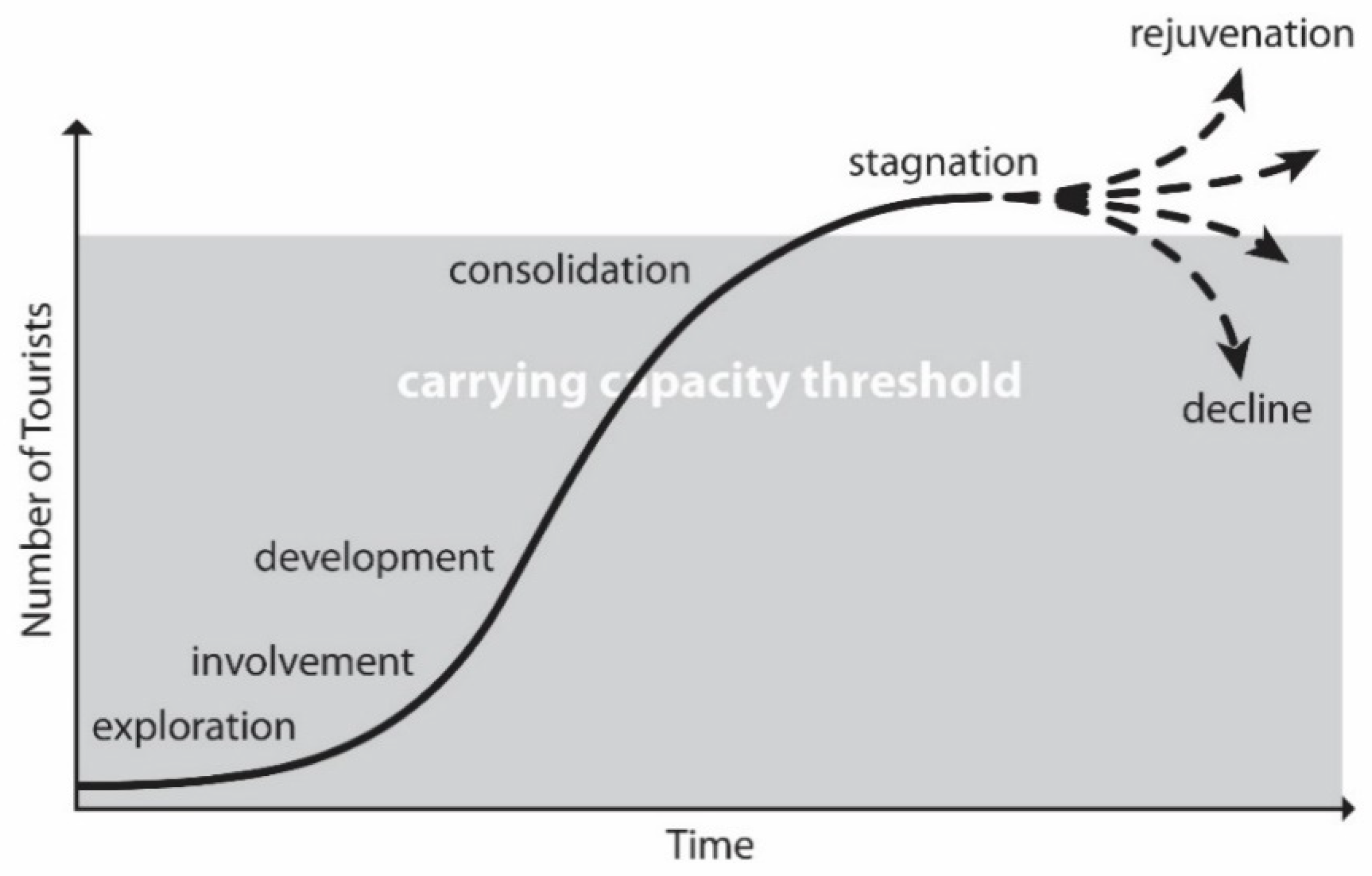This image showcases a detailed statistical chart illustrating the relationship between time and the number of tourists at a tourist location. The X-axis represents time, while the Y-axis indicates the number of tourists. The chart features a parabolic line that begins at 'exploration,' progresses through 'involvement,' 'development,' and 'consolidation,' eventually reaching a 'stagnation' phase. At stagnation, the line diverges into four potential paths: one arrow points upward toward 'rejuvenation,' another to the top right, one heading to the bottom right, and the last one descends sharply, signifying 'decline.' The graph is predominantly black with a gray background, and there's a significant light blue box in the center, likely highlighting the core data points. The 'carrying capacity threshold' is marked in white letters, crossing the consolidation phase. This visually contrasting and vividly annotated chart effectively conveys various possible tourist number trajectories over time.